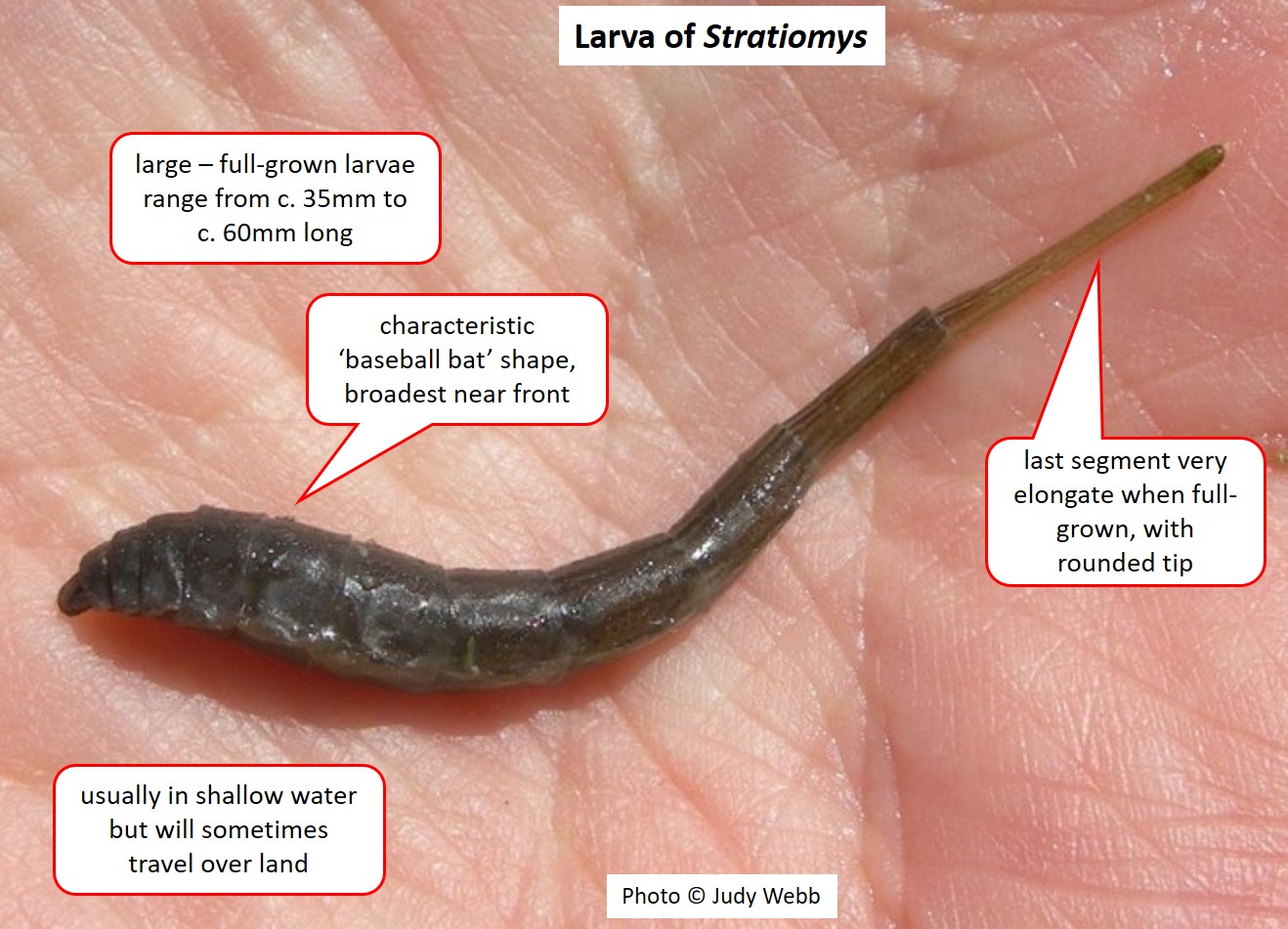This detailed image captures a zoomed-in view of a dark brown, slimy larva, identified as the larva of Stratiomys, lying in the palm of a fair-skinned person. The larva, approximately 35mm to 60mm long, exhibits a characteristic baseball bat shape, broadest near the front and tapering to a translucent brown, elongate segment with a rounded tip at the tail. The high-resolution photograph highlights the intricate creases and wrinkles of the person's palm. Several red-bordered, white-background labels with black text provide detailed information about the larva: “Large full-grown larvae range from circa 35mm to circa 60mm long,” “Characteristic baseball bat shape, broadest near front,” “Last segment very elongate when full-grown with rounded tip,” and “Usually in shallow water but will sometimes travel over land.” At the top of the image, a white box with black letters says "Larvae of Stratiomys." A rectangular white box at the bottom of the photo reads "Photo copyright Judy Webb." This informative image serves as both a scientific reference and an educational snapshot of the larva's morphology and habitat.